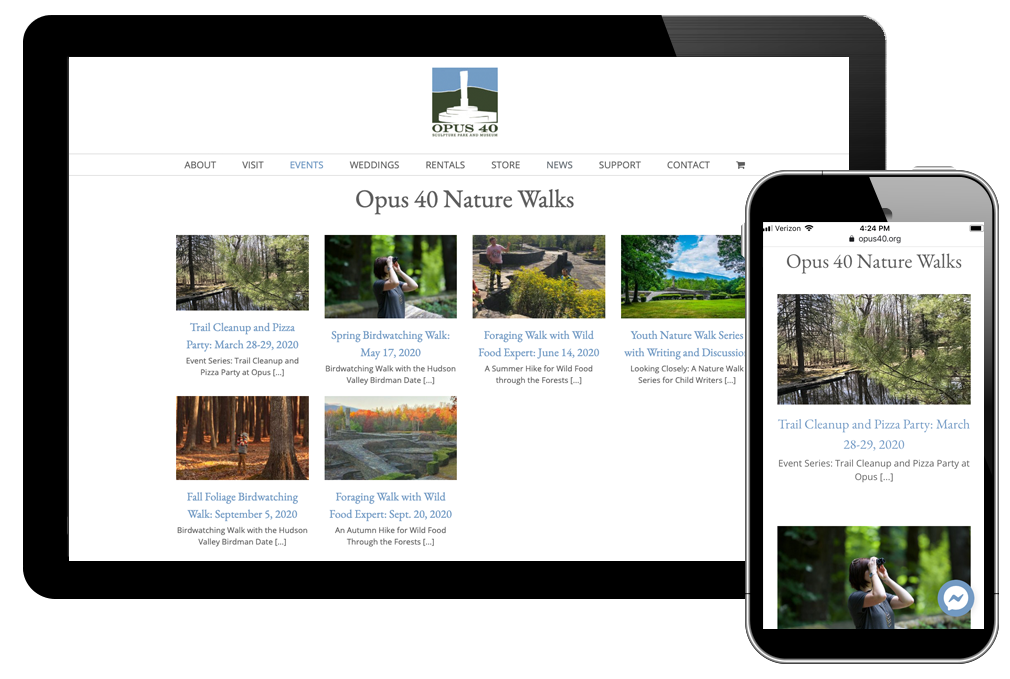Two images depict the Opus 40 Nature Walks website displayed on different devices: a tablet in landscape mode on the left and a smartphone on the right. The smartphone screen shows the website under the header "Open Nature Walks," with a timestamp of 4:24 p.m., Verizon network signal, and 90% battery life displayed at the top. A large landscape photo of a forest with a stream occupies the upper section, under which the text announces "Trail Cleanup and Pizza Party, March 28-29, 2020," followed by "Event Series." Below this, another landscape photo depicts a woman looking to her right through binoculars, her arms raised. 

The tablet version showcases the same content with additional elements. At the top, the Opus 40 logo is prominently displayed next to a strip of menu tabs: About, Visit, Events, Weddings, Rentals, Store, News, Support, and Contact. Underneath these tabs, the same website title "Opus 40 Nature Walks" is visible alongside six photograph thumbnails. The first two thumbnails mirror the images seen on the smartphone, highlighting the site's adaptation for different screen sizes.